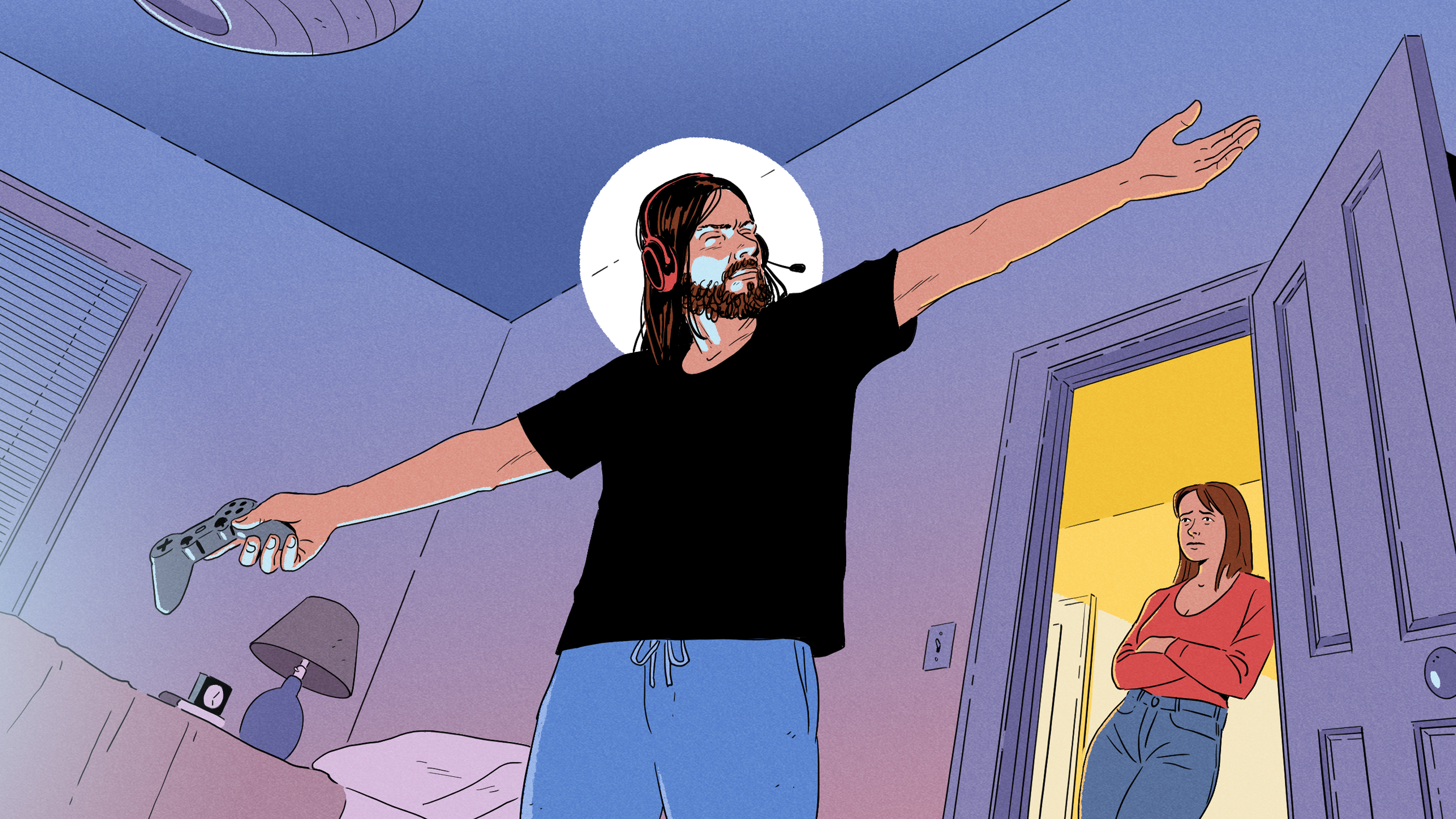This vibrant comic-style drawing captures a scene of a man in his bedroom, framed from a low angle as if viewed from the floor. The man, who has long hair and a beard reminiscent of Jesus, stands in the center with arms outstretched, clutching a video game controller in his right hand. He is adorned with a black shirt and blue drawstring pants, and wears a gaming headset with a microphone. A soft, pale yellow halo encircles his head, adding a divine aura to his focused demeanor. His eyes are closed, emphasizing his absorbed state.

To the left of the man, the room features a bed with a white pillow, a blue lamp with a purple shade on a nightstand, and a small black and white square detail, possibly another object or piece of decor. The walls and ceiling create a serene gradient from blue to a purplish hue at the bottom, enhancing the room's tranquil atmosphere.

In the background, an open doorway reveals a woman leaning against the doorframe with her arms crossed and a frown on her face. She has brown hair and is dressed in a red shirt and blue jeans, positioned against the backdrop of yellow walls. The scene blends everyday domesticity with an almost spiritual reverence for gaming.